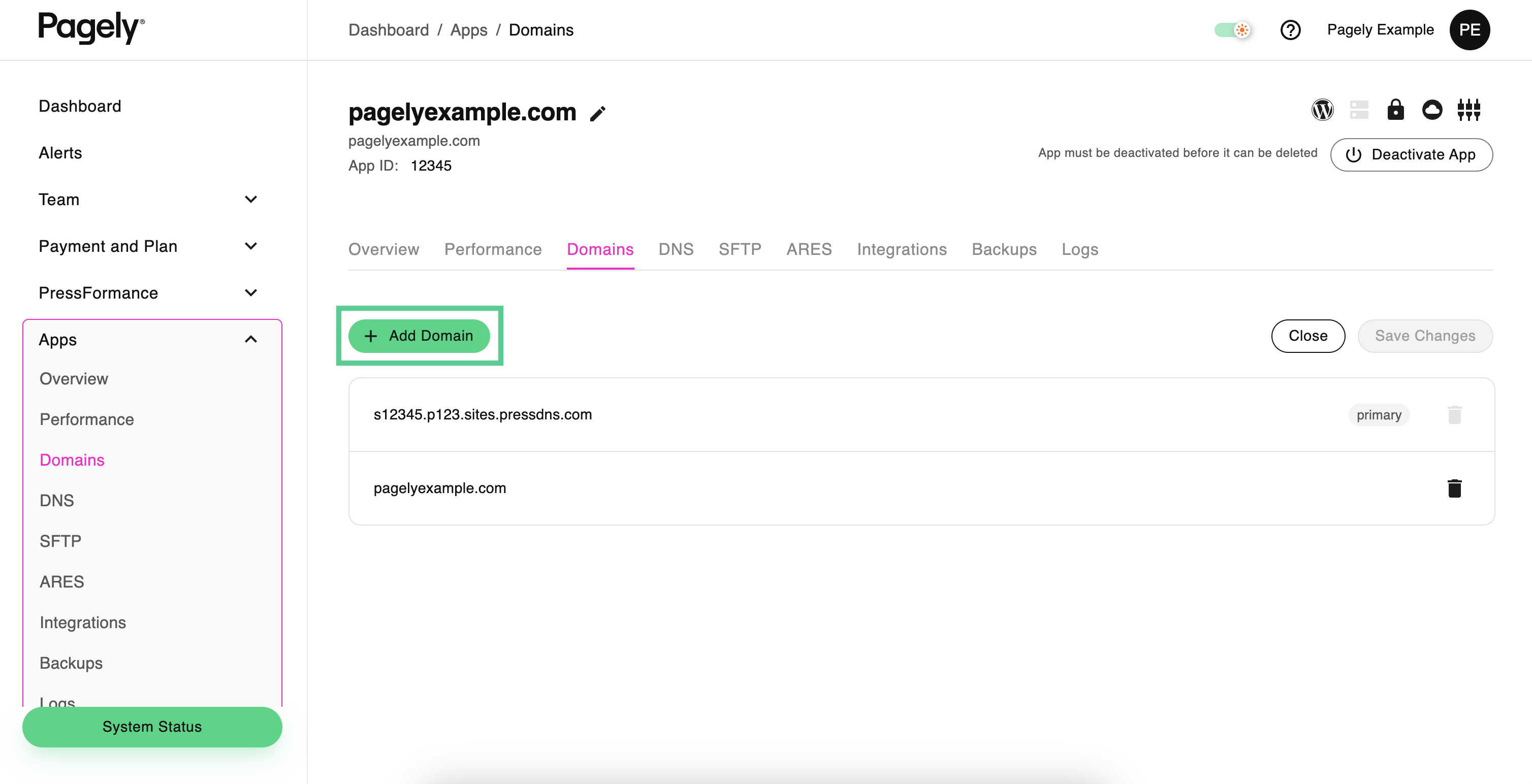The image is a screenshot from a Pagely web page, specifically displaying a section of their dashboard interface. At the top of the page, it is labeled "Pagely" with a navigation path indicated as "Dashboard / Apps / Domains." In the upper-right corner, it shows "Pagely Example," accompanied by a black circle containing the white letters "PE."

The left sidebar contains various menu options, including "Dashboard," "Alerts," "Team," "Payment and Plan," "PressFormance," "Apps," and under the "Apps" section, sub-categories such as "Overview," "Performance," "Domains," "DNS," "SFTP," "ARES," "Integrations," "Backups," and "Logs." At the bottom of the sidebar, there is a green oval button labeled "System Status." The "Apps" choice is outlined with a pink rectangle, and the "Domains" choice is highlighted in pink.

In the main content area of the page, the text "Pagely Example.com" is displayed alongside an app ID, "12345." Below this, the same navigation options from the sidebar—"Overview," "Performance," "Domains," "DNS," "SFTP," "ARES," "Integration," "Backups," and "Logs"—are shown again. A prominent green rectangle with a green oval inside contains the text "+ Add Domain." Below this button, the site "12345.p123.sites.pressdns.com" is listed, followed by "PagelyExample.com."